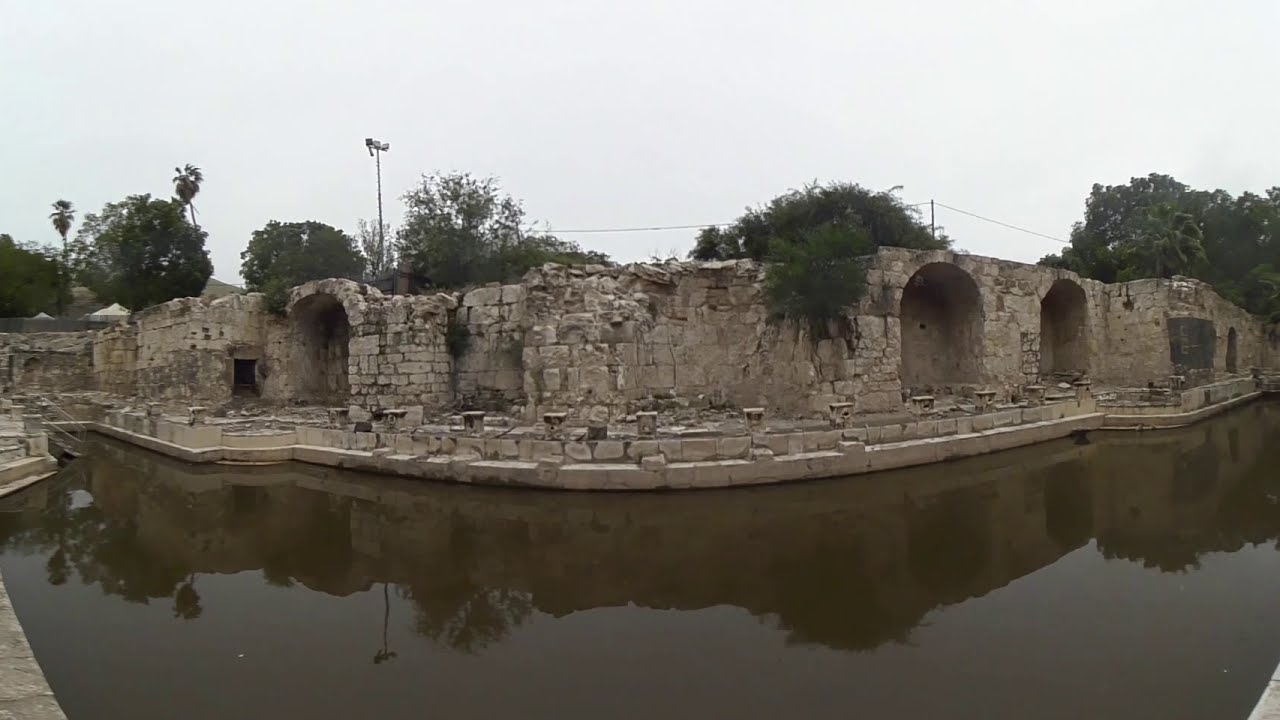The image captures an outdoor scene, likely a historic site or monument that has succumbed to time. Dominating the center of the image is a decaying stone wall, characterized by arched alcoves and crumbling rocks, that stretches from left to right. The wall appears to be the main feature and stands just above a stone walkway. Below the walkway, which has remnants that may have once functioned as benches or a fenced barrier, is a canal filled with murky brown water, suggesting neglect.

The bottom portion of the image frames this waterway, with patches of the stone wall dipping into the water on the lower left and right corners. On the far left, metal stairs descend into the canal, adding a layer of somber neglect to the scene.

A cluster of green trees trails above the stone wall, their branches slightly overhanging and blending into the desolate backdrop. Looming over all of this, the sky remains an overcast gray, enhancing the dreary, almost melancholic atmosphere of the photograph. To the left, in the distant background, a solitary light pole is visible, reinforcing the sense of abandonment.

The image’s overall tone is one of decay and desolation, perhaps capturing what once might have been a significant location—but now stands as a dilapidated, forgotten remnant of its past.